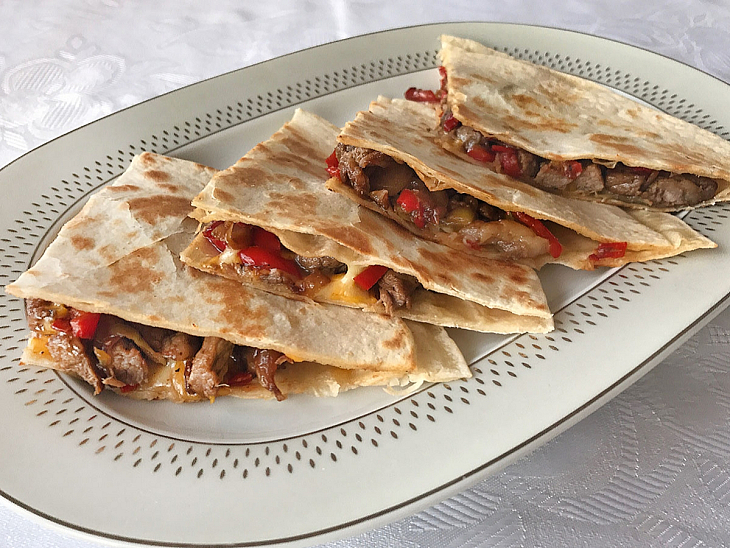The image is a close-up photograph showcasing a beautifully presented plate of quesadillas. These quesadillas are cut into four equal triangular pieces, revealing a savory filling of tender steak, melted cheese, and vibrant red peppers. The tortillas are perfectly browned, with a flaky, lightly crisped exterior. The presentation is meticulous, with the quesadilla pieces stacked neatly on top of one another, making it easy to see the delicious fillings inside. They are served on an elongated, oval-shaped white platter featuring a decorative silver border embellished with silver dots and a black outline. This elegant platter rests on a pristine white tablecloth, enhancing the overall sophisticated and appetizing presentation of the dish.